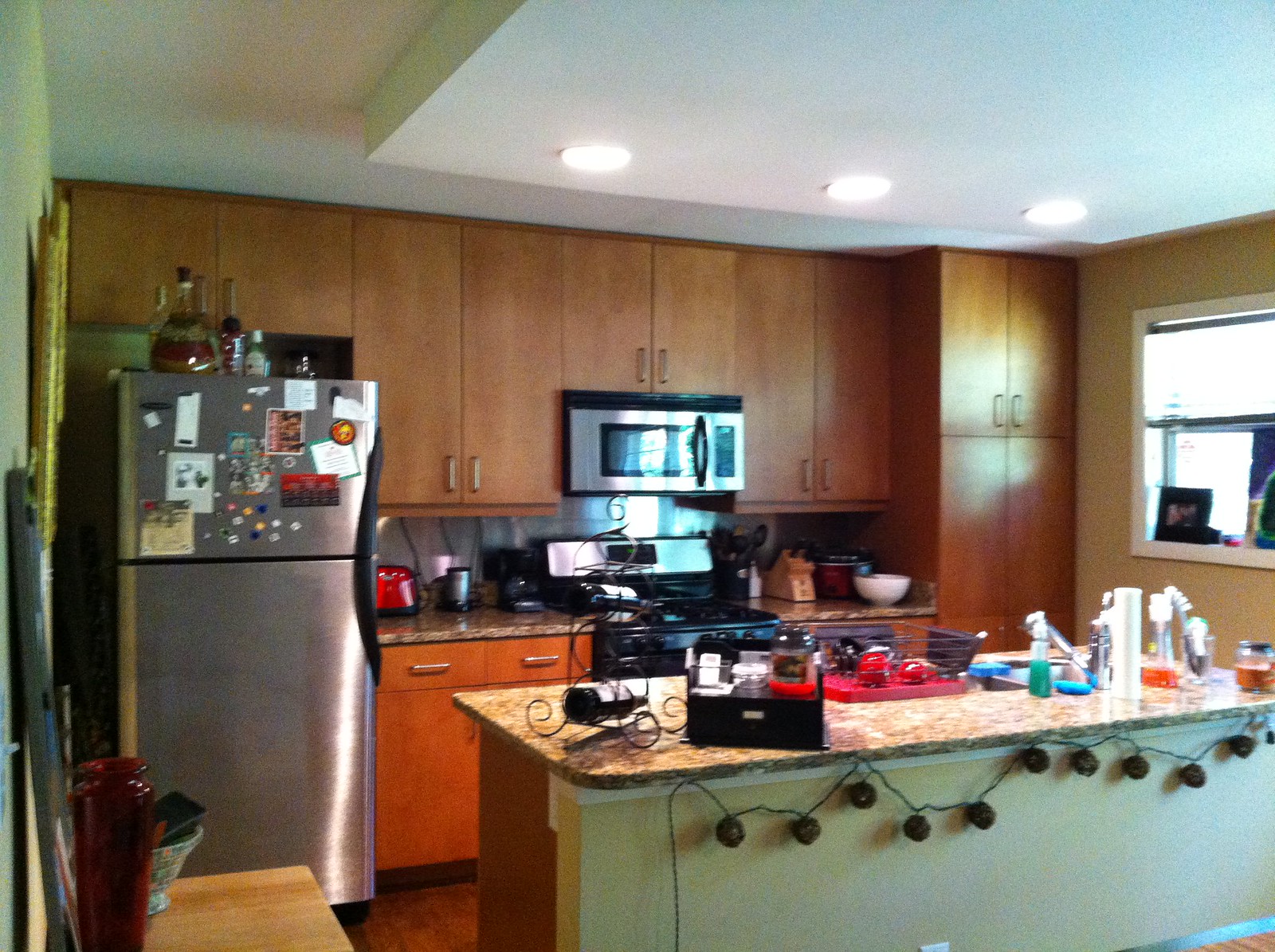A cozy kitchen with a small island takes center stage, featuring a variety of items that reflect a well-used and loved space. The island is adorned with a wine rack, a place for dishes, a sink equipped with a soap dispenser, and various miscellaneous kitchen items including a paper towel roll. Hanging from the island is a whimsical string of lights or small ornaments, adding a touch of decoration. The backdrop of the kitchen is composed of numerous wooden cabinets, a stove, and a microwave. A window above the counter displays picture frames on its sill, bringing a personal touch to the room.

The kitchen has ample counter space, populated with essential cooking tools such as knives, a white bowl, and a red toaster. A stainless steel refrigerator stands to one side, adorned with bottles and other liquids on its top. Adding to the room's charm is a wooden table that holds a striking red vase. A bulletin board with picture frames hangs on the wall, displaying photos or memories. The overall aesthetic of the kitchen is warm, with predominantly wooden elements, a green-painted island front, and a yellow-hued wall, creating a vibrant and inviting atmosphere.